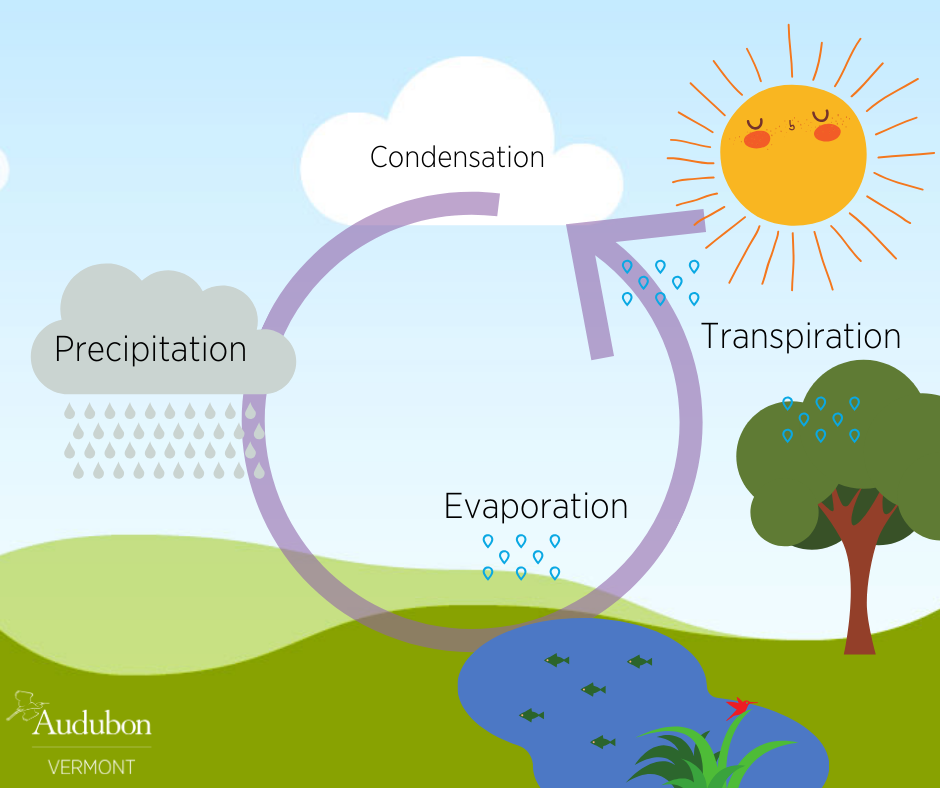This illustration demonstrates the water cycle, showcasing key processes such as condensation, precipitation, evaporation, and transpiration in a detailed and engaging manner. At the top, a white cloud labeled "condensation" floats in a light pastel baby blue sky, with a gray cloud to the left marked "precipitation" releasing gray raindrops. Beneath these clouds, there's a lush landscape featuring patches of green land, a vividly blue pond with a green plant and a pair of green fish, and a prominent tree with a brown trunk and green treetop marked "transpiration" at its top. A red flower blooms from the green plant in the foreground beside the pond, adding a splash of color. A series of blue teardrop-shaped bubbles rise labeled "evaporation," representing water moving from the pond back to the sky. A continuous purple arrow connects each element: starting from the white condensation cloud, moving to the gray precipitation cloud, down to the pond, across the tree, and looping back up to the white cloud. Completing the scene, a cheerful yellow cartoon sun with a cute face shines in the top right corner, underlining the illustration's kid-friendly design. In the bottom left corner, the text "Audubon" appears in white, with "Vermont" situated just below it.